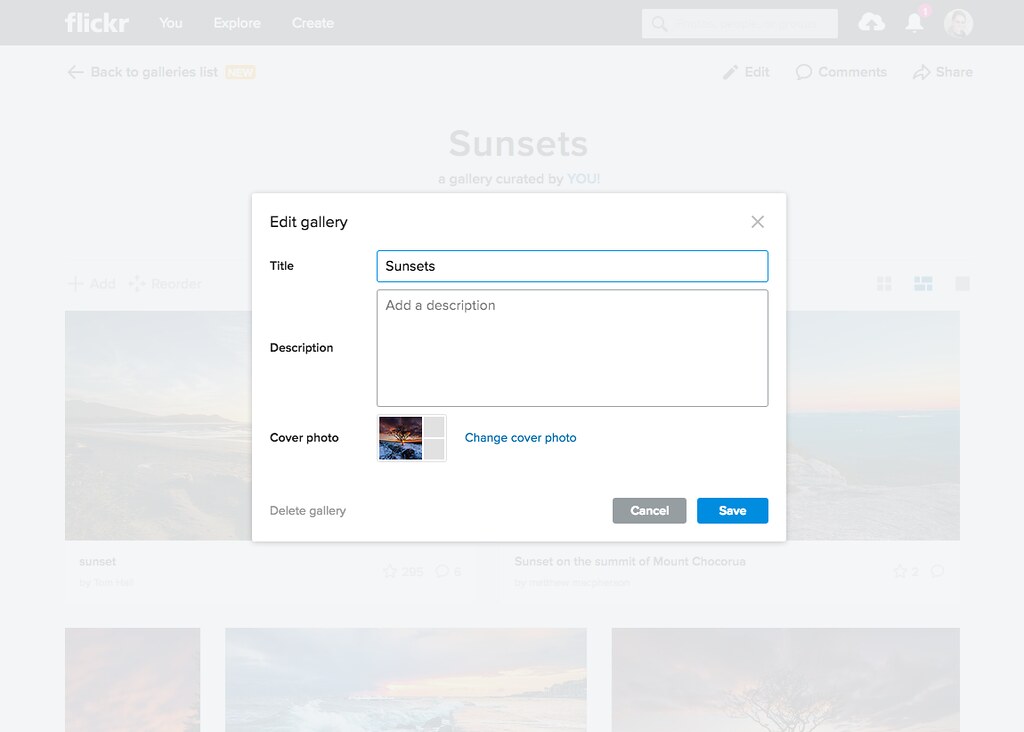This image is a screenshot from Flickr, featuring a grayed-out webpage with a central pop-up box titled "Edit Gallery". The pop-up has a clean white background and is divided into three primary sections: 

1. **Title Section**: On the left, it is labeled "Title" with an adjacent text bar outlined in blue containing the word "Sunset". 
2. **Description Section**: Below the title, it is marked "Description". Here, there is a sizeable text box to type in a description for the gallery. 
3. **Cover Photo Section**: The third section is for the cover photo. This section includes two small preview templates, with a blue "Change Cover Photo" link to the right.

Along the bottom of the pop-up box, on the left side, there is a small gray text option to "Delete Gallery". On the bottom right, there are two buttons: a gray "Cancel" button and a blue "Save" button. Additionally, an "X" at the top right corner allows users to close the pop-up.

In the background, the blurred and grayed-out Flickr page is seemingly about "Sunset", offering a subtle context to the pop-up's content.